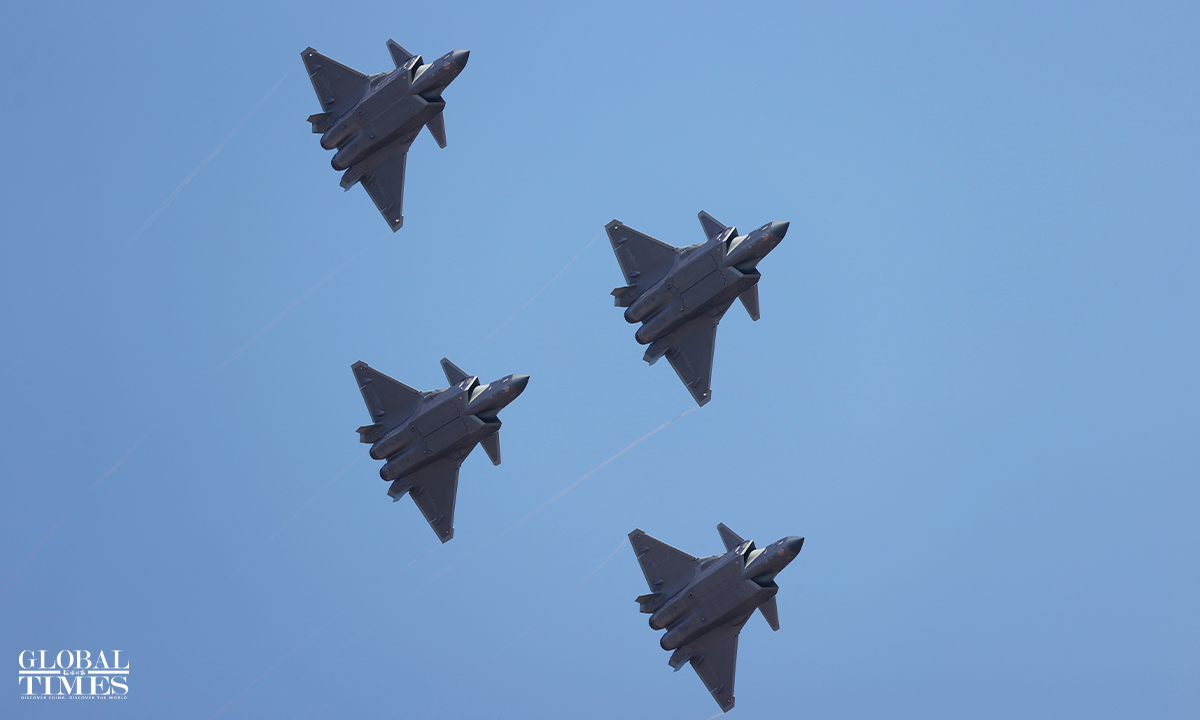The image captures five identical military fighter jets flying in perfect unison against a backdrop of clear, blue sky with not a cloud in sight. The jets are arranged in a distinct formation, starting from the bottom middle of the photograph and ascending towards the top left. The photograph, likely taken from the ground, offers a view of the jets' undersides as they perform at high speed, invoking the precision of an air show display. In the bottom left-hand corner, the text "GLOBAL TIMES" is prominently displayed in white, capital letters, suggesting that this high-quality horizontal image was featured in a publication.